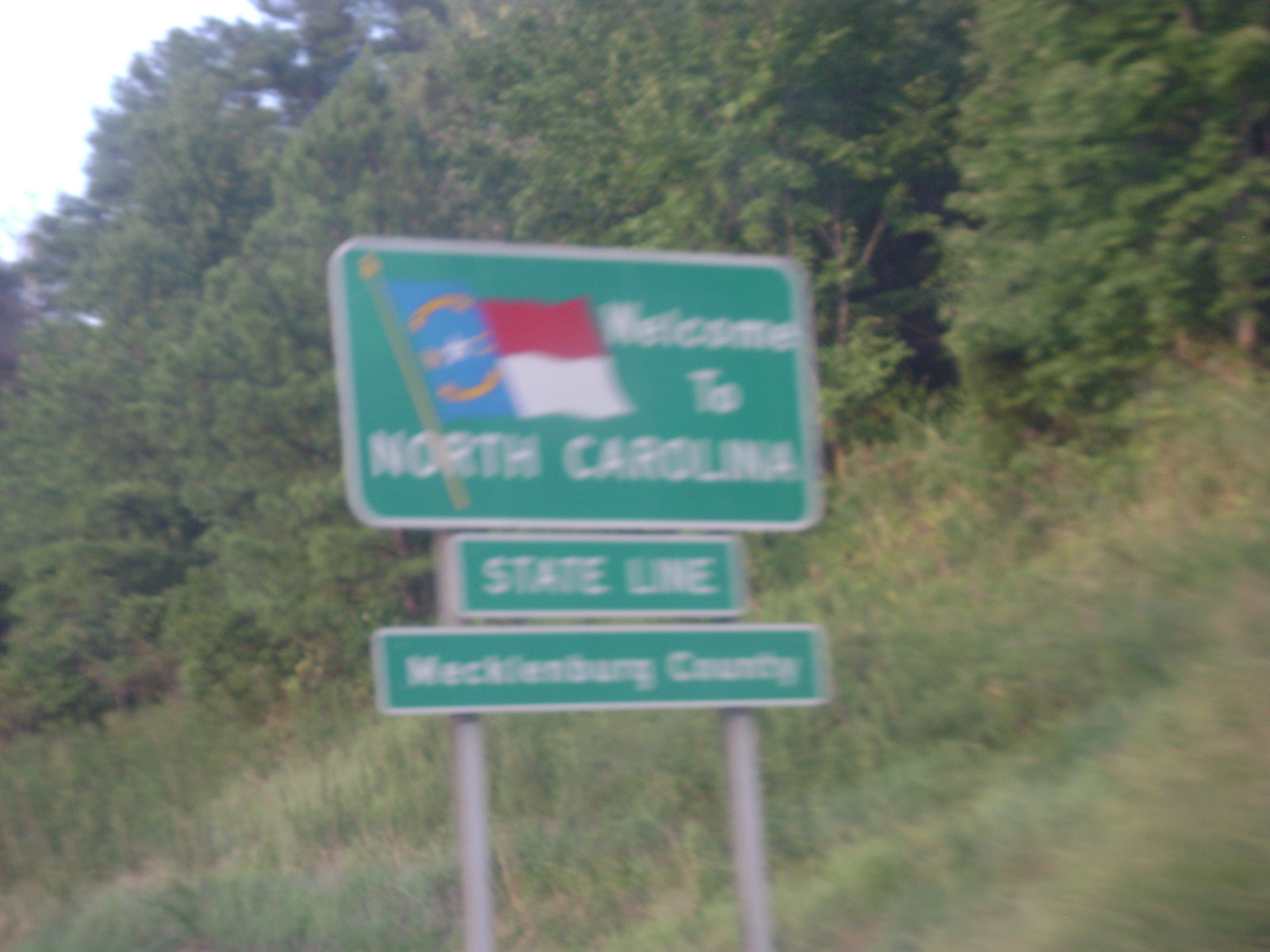The image depicts a series of traditional green traffic signs on the side of the road, held up by two silver posts against a backdrop of trees and grass. The top sign is a rectangular green sign with rounded edges and white text that spells out, "WELCOME TO NORTH CAROLINA," with the North Carolina state flag in the top left corner. The flag is divided vertically, with a blue half featuring two gold arrows forming a circle around a white and gold star, and a red and white strip on the right half. Below this, a smaller rectangular green sign reads "STATE LINE" in white font. The lowest sign, slightly longer, also has white text and declares "MECKLENBURG COUNTY." Despite the overall quality being noted as blurry, the detailed arrangement and content of the signs remain discernible.